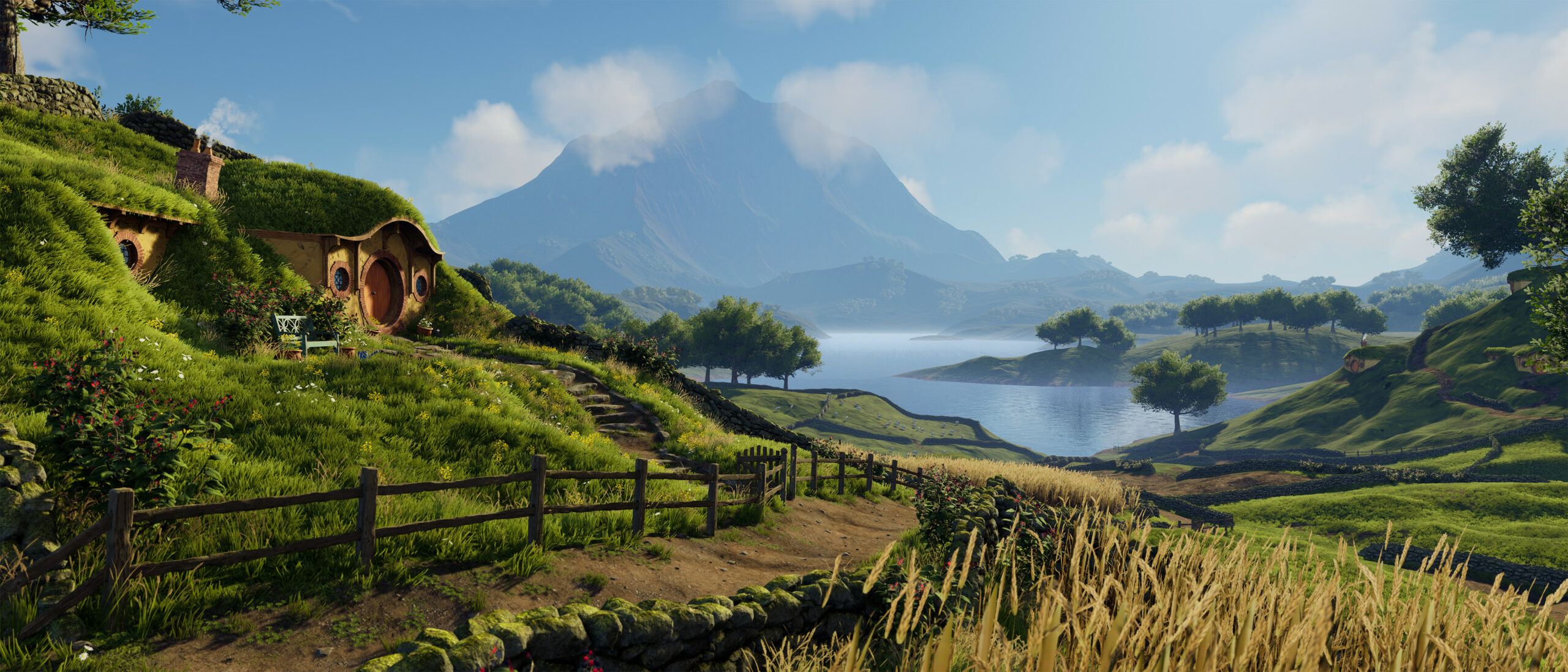This detailed painting captures a serene countryside scene. On the right side, there's a gently sloping hill at about a 45-degree angle, lush with green grass and topped by a large tree. Moving to the foreground, the landscape transitions into rolling grass alongside stalks of brown-white wheat, situated about an inch from the bottom of the image. A dirt pathway begins from the bottom left corner and snakes rightward toward the middle before turning left into a small walkway with barely noticeable stairs. Flanking the pathway is a sturdy wooden fence, behind which lies a slightly inclined grassy hill.

Nestled into this hill is a quaint house, blending harmoniously with the natural surroundings. The house, light brown with brown trim, features a distinctive circular front door of a dark brown hue, flanked by two windows. A roof covered in grass slopes gently upward and to the left, and from beneath the grassy cover, a chimney protrudes. Additionally, a bench is positioned in front of the house, offering a peaceful view of the landscape.

In the background, the sky is a clear blue, adorned with wispy clouds. Dominating the center is the outline of a giant mountain, cascading down into a shimmering lake. The lake boasts a small, tree-covered island, enhancing the idyllic setting. Green hills and a scattering of vibrant flowers dot the right side of the image, further enriched by the presence of additional trees. Capturing the essence of springtime, this artwork combines natural beauty with rustic charm, creating a picturesque rural vista.